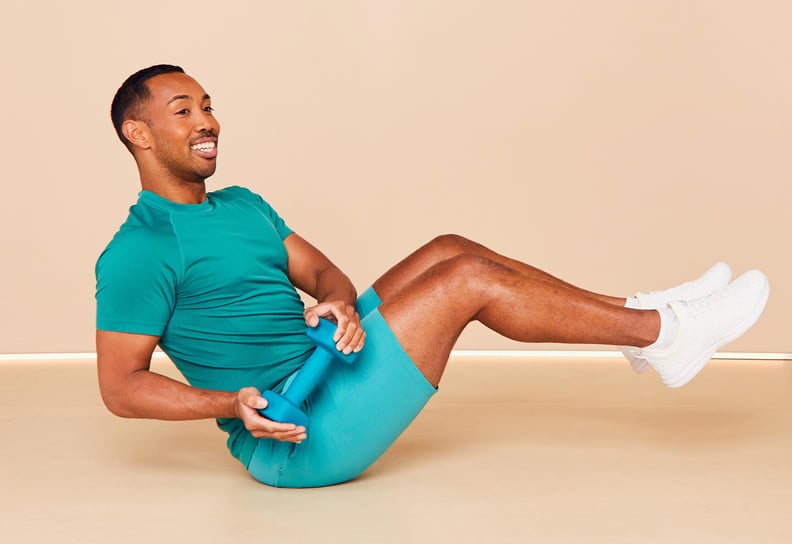The image features a muscular, light-brown-skinned, young African-American man likely in his 30s, engaged in an exercise routine. He has very short black hair and noticeable stubble on his face that doesn't quite form a full beard. His face is captured in a three-quarters view as he smiles. Dressed in a dark green teal or aqua-colored short sleeve t-shirt and matching tight workout shorts, he complements his outfit with white sneakers and socks. 

Seated upright on a tan floor, which is seamlessly connected to a similarly colored wall by a white horizontal line, the man is performing a twisting exercise. His legs are raised and bent, hovering above the ground as he twists to his right side, holding a teal-colored barbell that weighs approximately 10-15 pounds. His poised posture indicates he's engaging multiple muscle groups to maintain stability. The overall scene captures his dedication and cheerful disposition while working out.